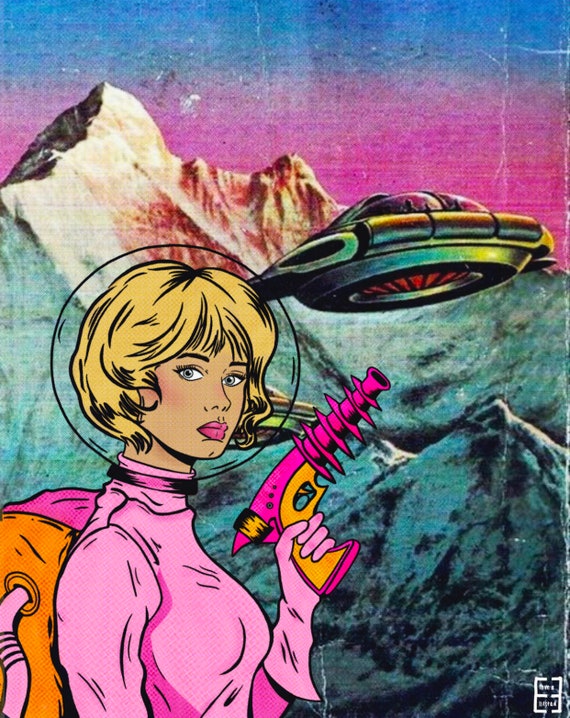This vertically aligned rectangular animated image, resembling a retro sci-fi poster, features a detailed illustration of a galactic girl on the left side. The woman has short styled blonde hair, green eyes, and is adorned with pink lipstick and pink blush. She gazes directly at the viewer with an expression of determined calmness. Her clear glass helmet, resembling a fishbowl, encircles her head without any visible attachments, accentuating her cartoon-like features and comic book style.

She is clad entirely in an all-pink space suit, including pink gloves, and holds a brightly colored 50s style ray gun with an orange handle in her left hand. On her back, she carries an oxygen tank with a pink hose, predominantly pink with an orange section on the side. 

To the right of the woman, a spaceship occupies the middle to upper portion of the image. This oval-shaped flying saucer, green and blue in color with a domed window, appears to have occupants visible inside. Below the saucer, a red circle featuring various ridged designs suggests some form of propulsion or energy beam.

The background sets the scene on another planet, likely Mars, characterized by a striking sky that transitions from blue at the top to bright pink below. In front of this colorful sky, a mountain range stretches across the image. These mountains are predominantly tan with some red highlights on the ridges, eventually blending into gray at the base, indicating areas cast in shadow. The overall art piece exquisitely melds elements of collage, different mediums, and pop art styles, enhanced by the presence of wrinkles or cracks in the poster-like material, adding a vintage touch.